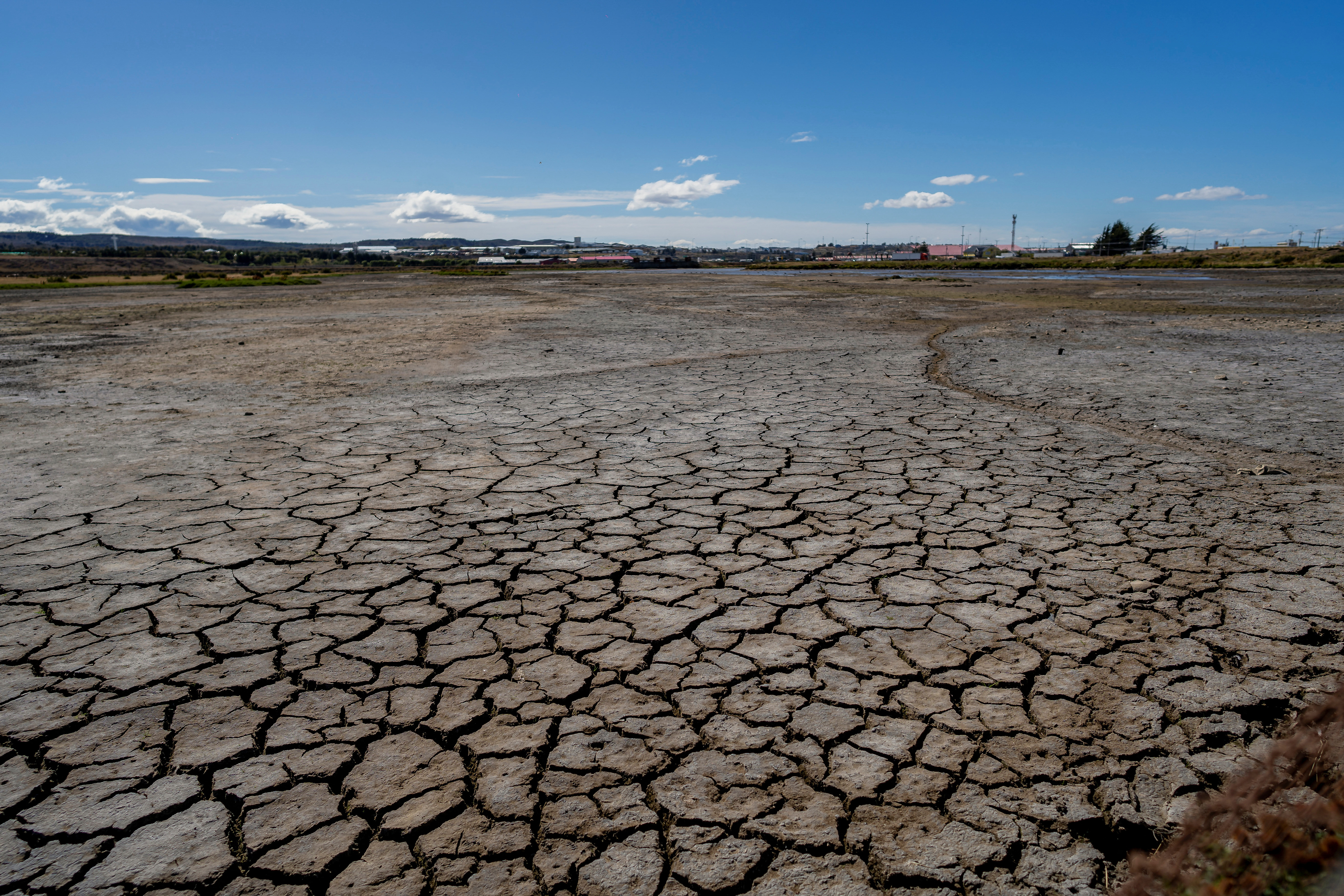The image captures a desolate, extremely dry area with deeply cracked dirt in the foreground, suggesting rapid evaporation of water or a prolonged period of drought. Minimal vegetation is present, with patches of brown and almost no green, highlighting the arid conditions. To the right, there is a hint of a trail, possibly from a vehicle, leading towards the distance. About 100 feet away, there appears to be a glimmer of water, indicating a nearby but not easily accessible water source. Beyond this point, the landscape transitions with trees and some buildings, and in the farthest horizon, mountains loom, adding depth to the scenery. The sky above is a striking blue with a few scattered, fluffy white clouds, creating a stark contrast to the parched earth below. The overall setting suggests a desert-like region, possibly reminiscent of areas in Nevada, Arizona, or New Mexico, characterized by intense dryness and rugged terrain.